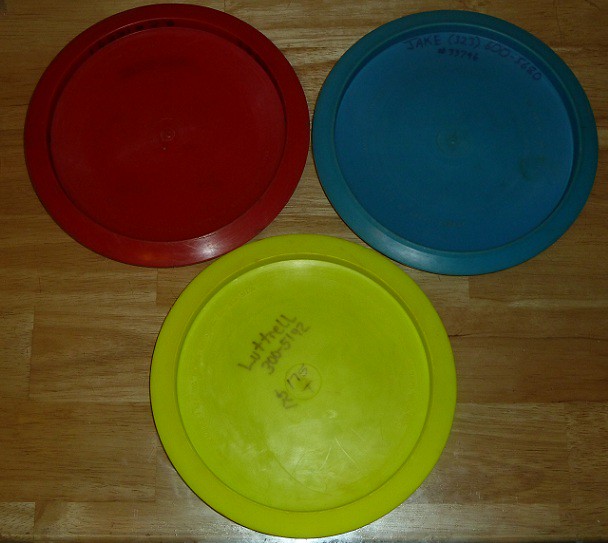This image, taken from a top-down perspective, captures three circular discs that resemble Frisbee golf discs, arranged in a triangle pattern on a light brown, wooden tabletop made of various long rectangular pieces of wood with subtle color variations. In the top left, there is a deep red disc; to its right, a deep blue disc with the name "Jake" and a partially obscured phone number inscribed on it. At the bottom center is a bright yellow disc displaying the name "Luttrell" and the phone number "300-5192" along with additional markings, including "175" on the left and a possible "175+" at the top. The photograph, likely taken indoors, showcases these vibrantly colored discs prominently within the frame, set against the rustic, farmhouse-style tabletop.